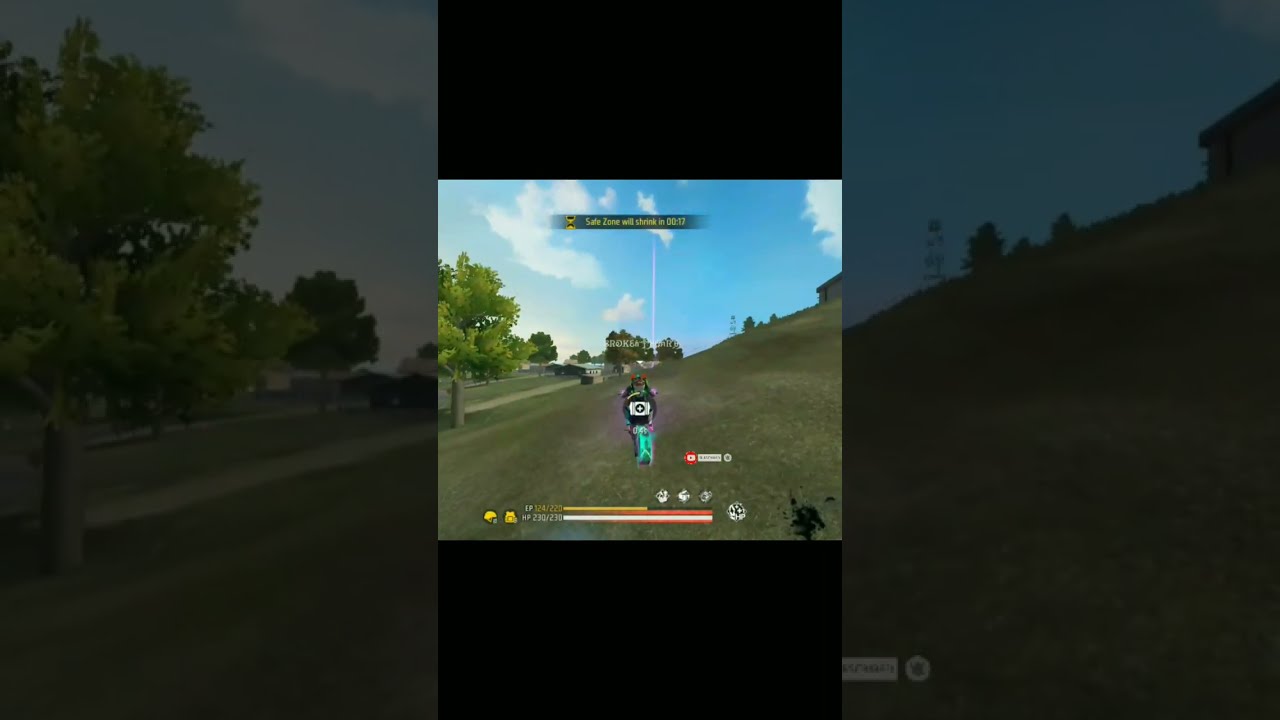The image is a screenshot from a video game, characterized by a dual-layered presentation. The central portion features a small, square clip of the game, which appears in clear focus against a darker, blurry overlay of the same scene in the background. The main image within the square shows a person in dark green clothing riding a teal motorbike on a steep, grassy hillside tilted at about 40 degrees. The grass has a muted, darker hue. This hillside seems to level out into a road on the left side, bordered by trees. The sky above is a vibrant blue with pixelated clouds. 

Various interface elements are present, including indiscernible yellow text above the character's head and progress bars in yellow, white, and red at the bottom, suggesting in-game stats or data. The overall composition is detailed, with trees on the left-center side and a cyan sky providing depth to the scene. All text in the image, including additional data at the top and bottom of the screenshot, remains blurry and unclear.